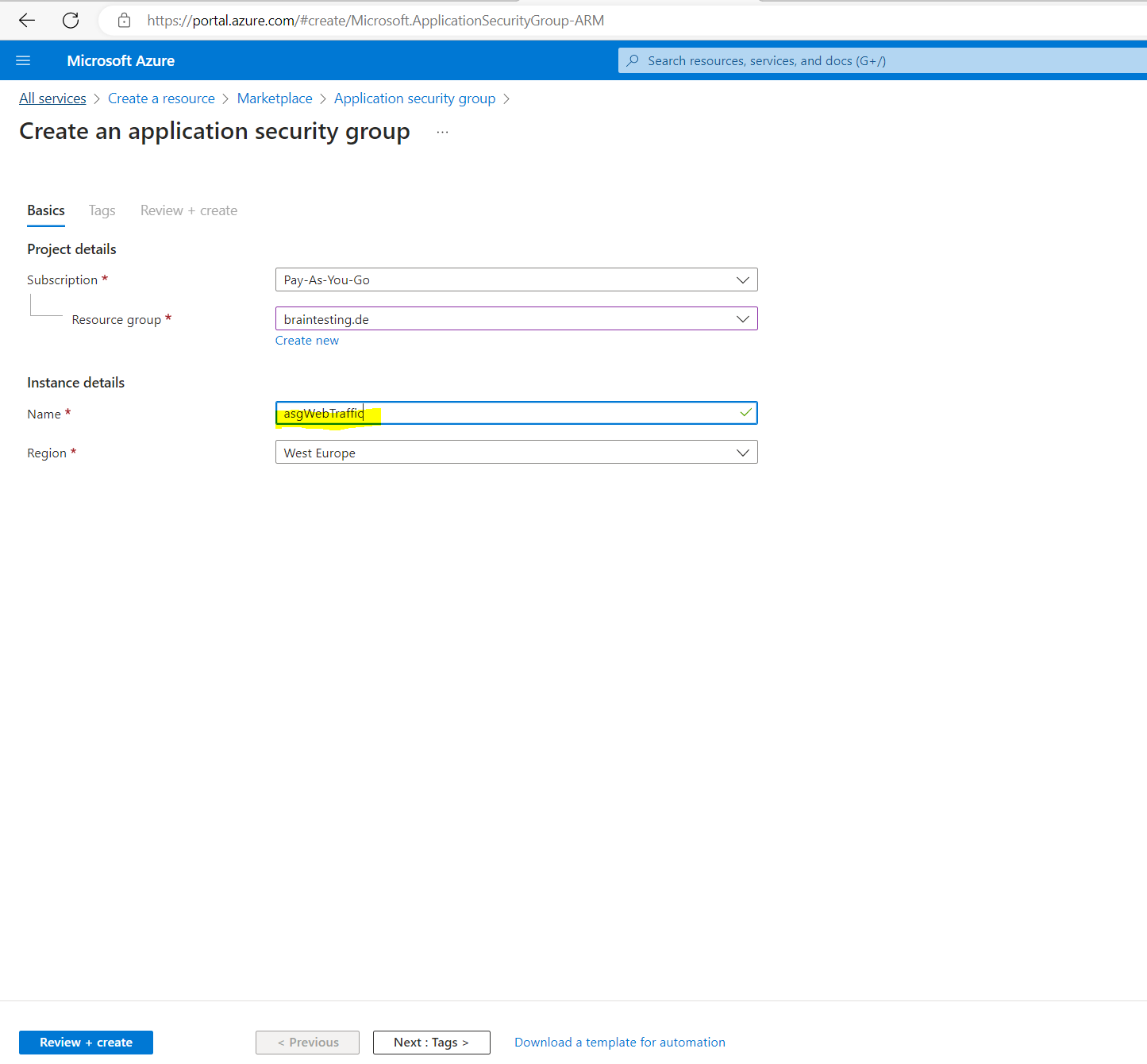The image depicts a detailed screenshot of the Microsoft Azure portal. At the top, a thin gray horizontal line spans the width of the screen. Beneath this line, the background is also gray. On the left side of the image, a black arrow points to the left, followed by another black arrow within a circular icon indicating a refresh action.

In the central portion, there is a white oval where users can type the website URL. The URL within this oval starts with "https" in dark gray, followed by "portal.azure.com" in black, and continues with "/#create/Microsoft.applicationSecurityGroup-ARM" in gray. 

Directly below, a blue rectangle stretches across the screen. On the left of this rectangle are three horizontal white lines indicating a menu. The words "Microsoft Azure" are displayed in white towards the center-right of the rectangle. Further to the right, but not fully visible, is a light blue rectangle with a blue magnifying glass icon next to the text. The visible part of the text reads "resources. Search resources, commerce services, and docs."

Underneath this header, there are several blue tabs, starting with "All services," which is underlined in a darker blue to indicate it is the active tab. The subsequent tabs include "Create a resource," "Marketplace," and "Application security group."

In the main section of the image, the text "Create an application security group" is prominently displayed in black. Below are several sections labeled "Basics," "Tags," "Review + create," featuring project details such as "Description," "Resource group," "Instance details," "Name," and "Region."